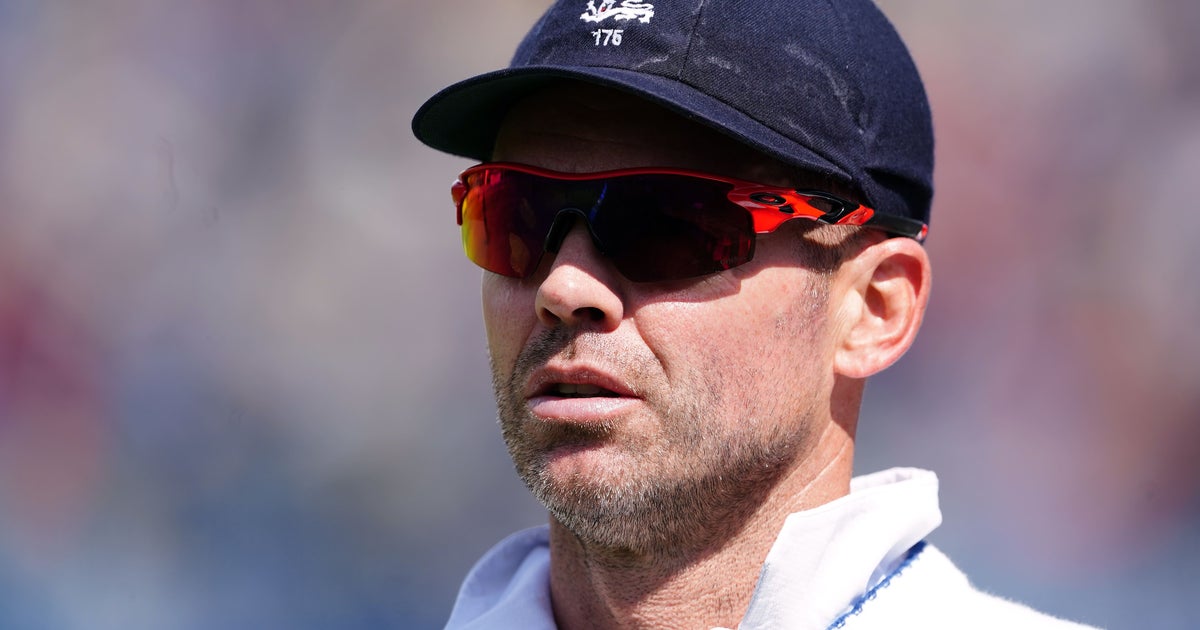The image depicts a close-up portrait of a white man in his 30s or 40s, wearing a navy blue baseball cap adorned with white embroidery that reads "175" or "176." He sports red and black sunglasses with very dark lenses that obscure his eyes, and his right ear is visible from the photograph's angle. His facial hair consists of a few days' stubble, giving him a short beard or 5 o'clock shadow look. He is wearing a white polo shirt with a blue trim under a slightly popped-up collar. The man's mouth is partially open, revealing some of his teeth, as he gazes off into the distance. The background is blurred, featuring a mix of blue, purple, and gray hues, making the man's detailed features and clothing the focal point of the image.